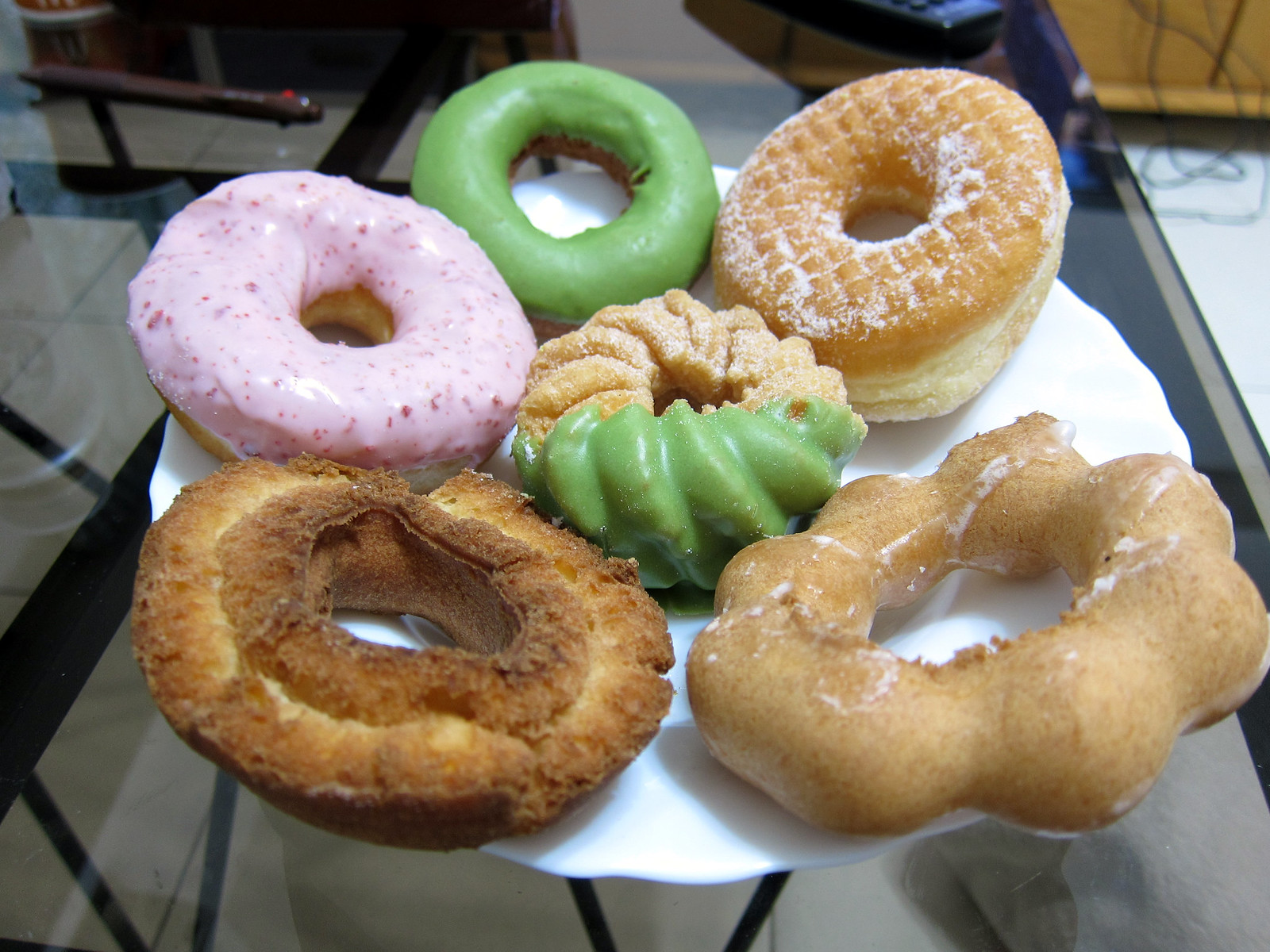This photograph showcases a white plate with elegantly curved edges, holding six distinct types of doughnuts, arranged in a circular pattern around the edge with one in the center. The plate, situated on a glass table with visible black metal boning and a hint of a TV remote control in the background, features an assortment of pastries: a central cruller doughnut partially glazed with green icing, a pink iced yeast doughnut presumed to be strawberry flavored, a chocolate cake doughnut frosted with green icing, a plain cruller-like doughnut with a slightly dry, bread-like texture, a traditional original glazed doughnut, and another with a light sprinkle of white sugar. The table setting suggests an office environment, inferred from the visible cabling under the glass surface.